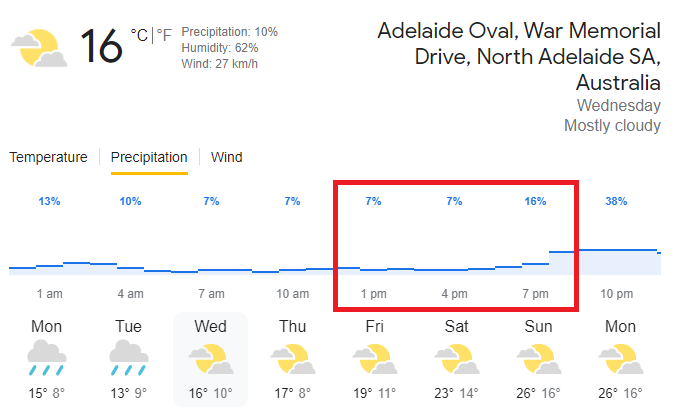The image features a weather forecast layout on a white background. At the top, there's an icon of a sun partially covered by two gray clouds, indicating a temperature of 16 degrees Celsius. Next to it, additional weather details are provided: 10 percent chance of precipitation, 62 percent humidity, and wind speeds of 27 kilometers per hour. 

On the right side, the location is specified as Adelaide Oval War Memorial Drive, North Adelaide, SA, Australia. The forecast states it is a Wednesday with mostly cloudy weather conditions. Various weather parameters including temperature and precipitation are highlighted, with parts underlined in yellow to draw attention to specific details.

Spanning the top of the image, the forecast is presented for a week, from Monday to the following Monday. Percentages for precipitation are also given: Monday at 13 percent, Tuesday at 10 percent, Wednesday at 7 percent, Thursday at 7 percent. Notably, Friday, Saturday, and Sunday are outlined in red, showing precipitation rates of 7 percent, 7 percent, and 16 percent respectively, while the following Monday has a higher precipitation chance of 38 percent.

A blue graph with a red square highlights the specific times on Friday and Saturday (1 p.m., 4 p.m., and 7 p.m.). Further daily weather details show:
- Monday: Rain, 15 percent, and 8 percent
- Tuesday: Rain, 13 percent, and 9 percent
- Wednesday: Cloudy, 16 percent, and 10 percent
- Thursday: Cloudy, 17 percent, and 8 percent
- Friday: Cloudy, 19 percent, and 11 percent
- Saturday: Cloudy, 23 percent, and 14 percent
- Sunday: Cloudy, 26 percent, and 16 percent
- The following Monday: Cloudy, 26 percent, and 16 percent.